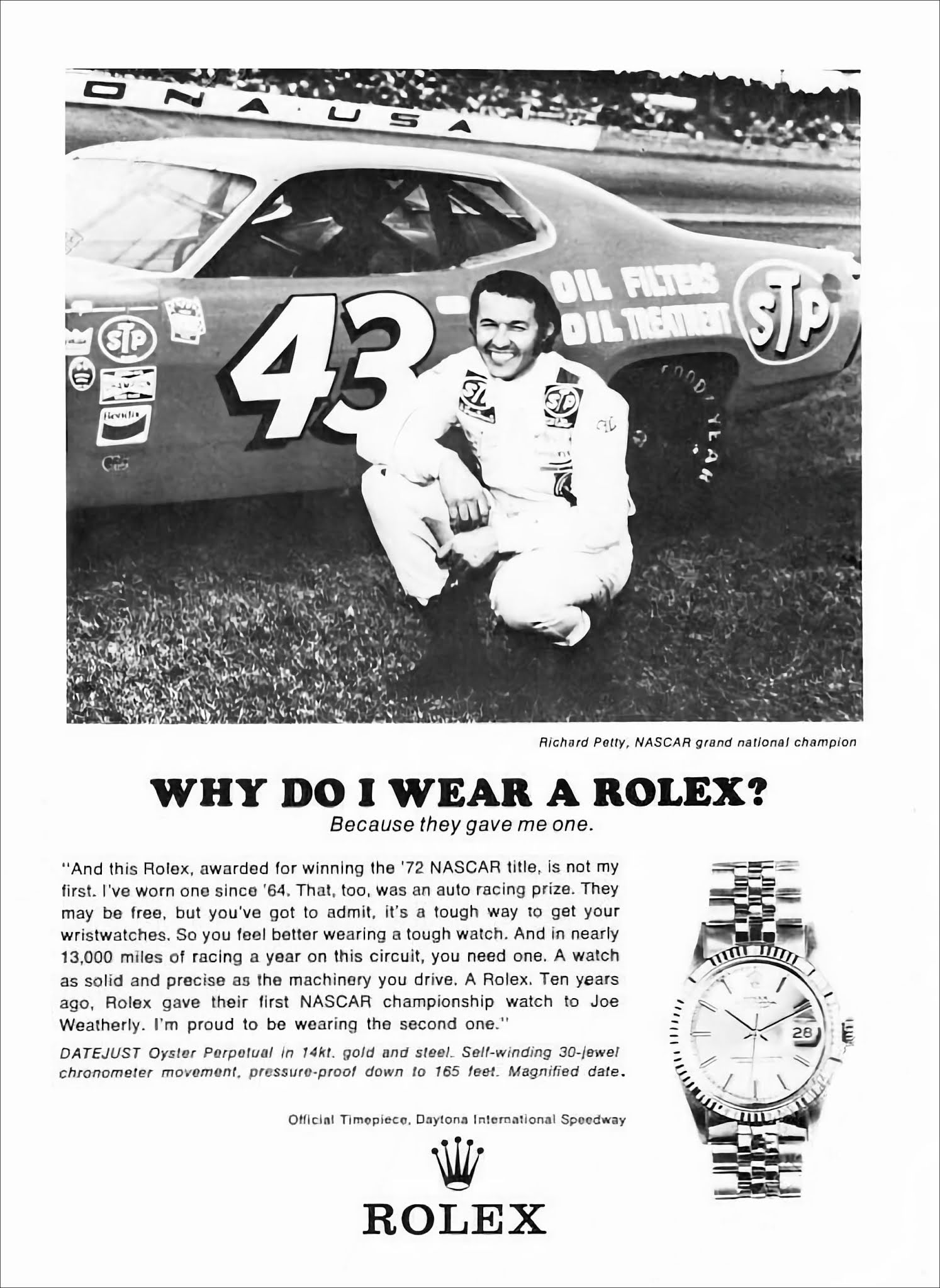This black-and-white advertisement from a race guide program features a young Richard Petty, NASCAR Grand National Champion, kneeling and smiling in front of his iconic number 43 race car. The car is adorned with various advertisements including the prominent STP logo as well as "oil filters" and "oil treatment" text. Richard Petty is also wearing a shirt with the STP motor oil markings. The background highlights the Daytona USA Speedway. The caption reads, "Why do I wear a Rolex? Because they gave me one." The ad elaborates that Petty won this Rolex for his 1972 NASCAR title, mentioning that he's worn a Rolex since 1964, thanks to previous racing prizes. The text notes that the first NASCAR champion to receive a Rolex was Joe Weatherly. The advertisement proudly showcases Rolex as the official timepiece of Daytona International Speedway, featuring an image of a Rolex watch with its iconic crown logo.